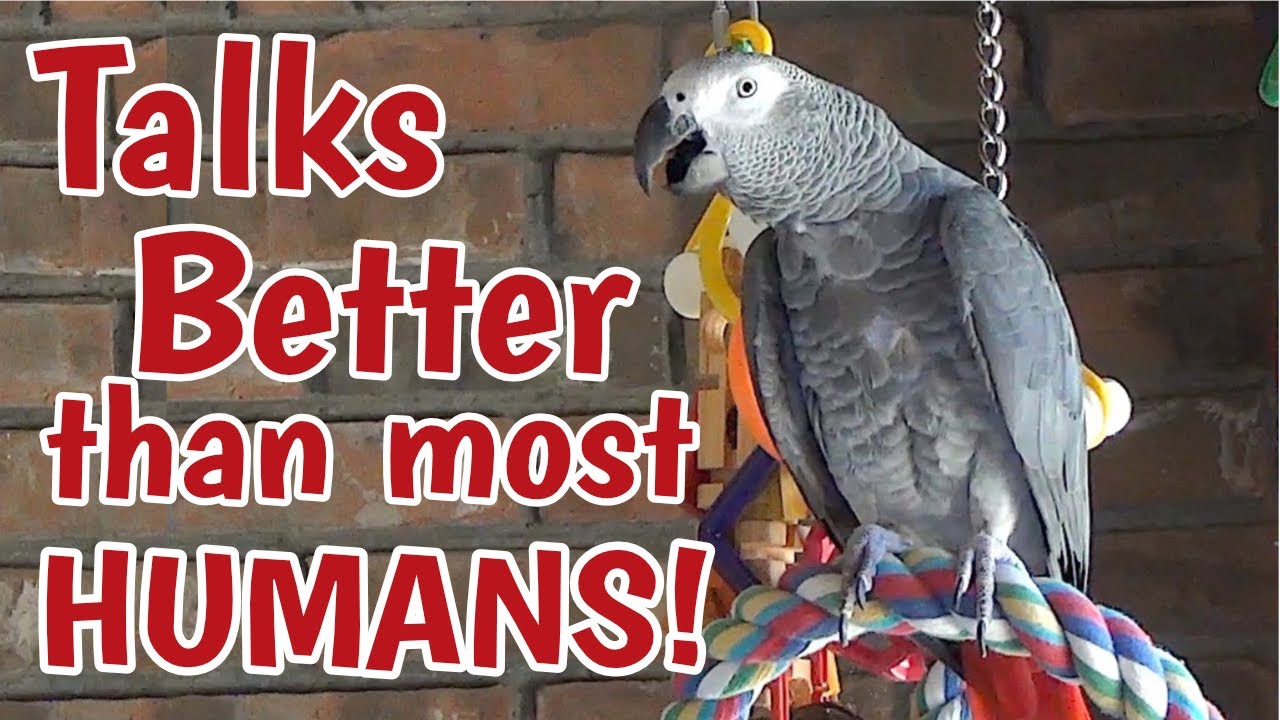This detailed image showcases a beautifully rendered African Gray Parrot, positioned on the right side of the scene. The bird is perched on a vividly colored braided rope, which hangs from a visible chain behind it. Accompanying the bird are various hanging toys, including wooden blocks and multicolored pieces in shades of yellow, orange, and blue. They are strung together with a carabiner, adding to the playful atmosphere. The background is a faded brick wall, giving the image a rustic, indoor setting. Above the parrot, a large, bold, deep red sans-serif font with a white outline proclaims, "Talks Better Than Most Humans!" The bird’s beak is slightly open as if in mid-conversation, and its posture appears relaxed, with its wings down, conveying a calm demeanor. The parrot is predominantly gray, with subtle hints of blue on its feet and a small blue patch visible on its chest. The overall composition and added text suggest a humorous and affectionate representation of the bird's impressive vocal abilities.